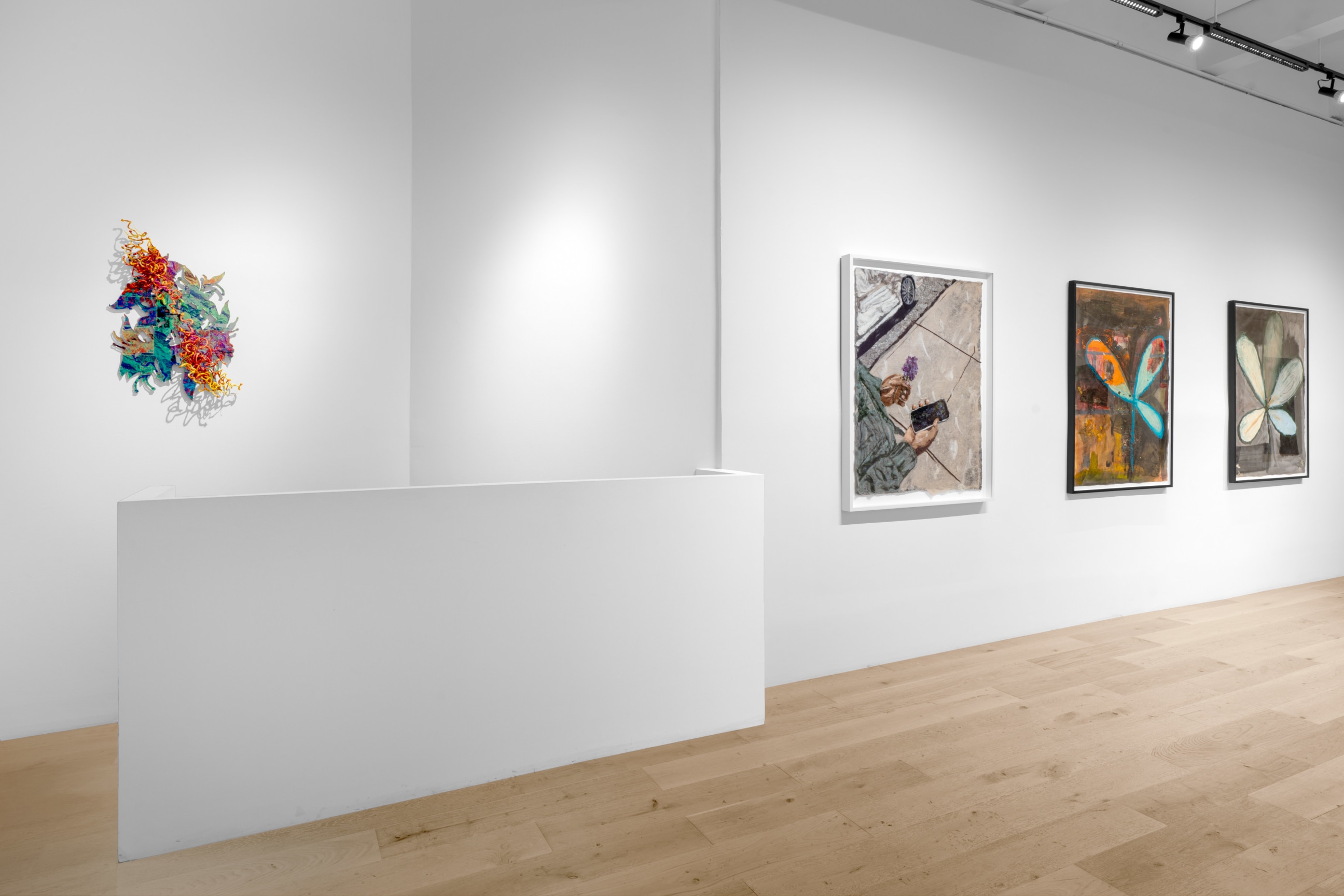This photograph captures the serene atmosphere of an art gallery featuring a harmonious blend of contemporary art pieces. The gallery is characterized by its multiple white walls running horizontally, all uniformly painted white. Central to the layout is a low, waist-high wall also painted white, which conceals a small cubby behind it.

On the left section of the gallery, an eye-catching abstract sculpture hangs on the wall. This vibrant piece is composed of various red, orange, blue, and yellow elements, arranged in a dynamic and visually engaging manner. Next to it, further to the right, a floral arrangement artwork is displayed. This piece features a mix of blue, pink, red, and light green colors, with intricate squiggly designs interwoven, giving the appearance of a delicate bouquet.

Dominating the right-hand side, three distinct paintings are showcased. The leftmost painting, set in a white frame, depicts a person holding a smartphone in one hand and a flower, possibly a purple lilac, in the other—a contemplative portrait blending technology and nature. The other two paintings, framed in black, present abstract forms reminiscent of dragonfly wings. The first features a combination of blues and oranges, while the second contrasts with a black and white palette, portraying white wings against a black or light gray background.

The gallery's ambiance is complemented by a light-colored hardwood floor, laid out in a plank pattern akin to laminate flooring. Above, the ceiling is adorned with black track lighting, providing focused illumination. Two black track lights are visible in the upper right corner of the photograph, ensuring each artwork is well-lit and highlighted to its best advantage.